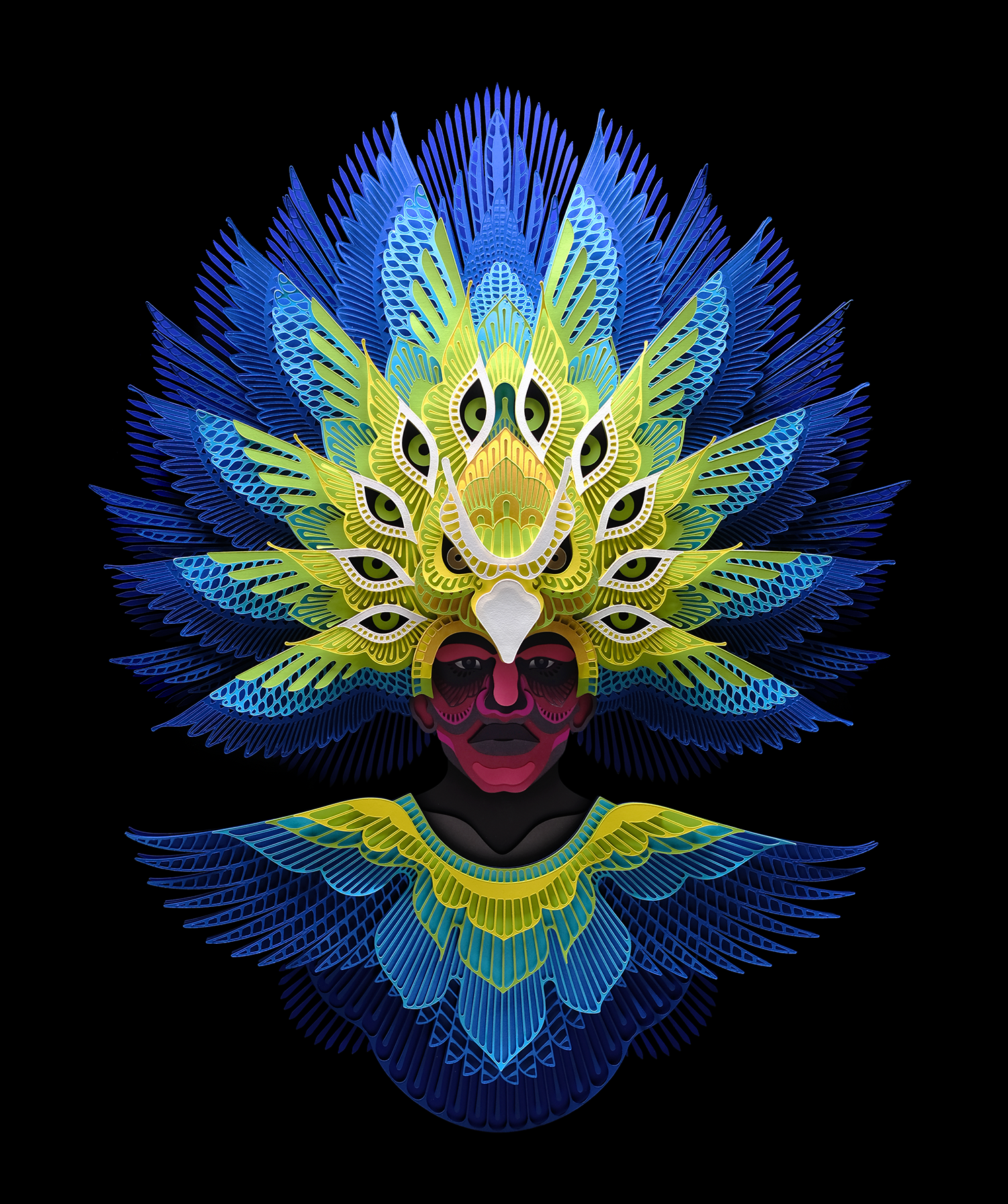This digital artwork features a striking central figure adorned with elaborate designs. The focal point is the face, painted with vibrant pink tones around the eyes and mouth, contrasted by a grey complexion that extends to the neck. The head is crowned with an intricate headdress resembling an ornate bird, with a golden piece arching from ear to ear across the forehead. The beak of the bird cascades between the eyes, flanked by symbols resembling eyes. The headdress's base color transitions from yellow to blue towards the feathered edges, echoing the wing-like patterns also found on the chest piece that covers the shoulders, mimicking shoulder pads. Additional blue and yellow patterns highlight the head and neck area. This figure, perceived as female, is richly adorned with a ceremonial outfit that evokes a peacock's grandeur and is depicted from the chest up against a stark black background, emphasizing its digital and animated origins.